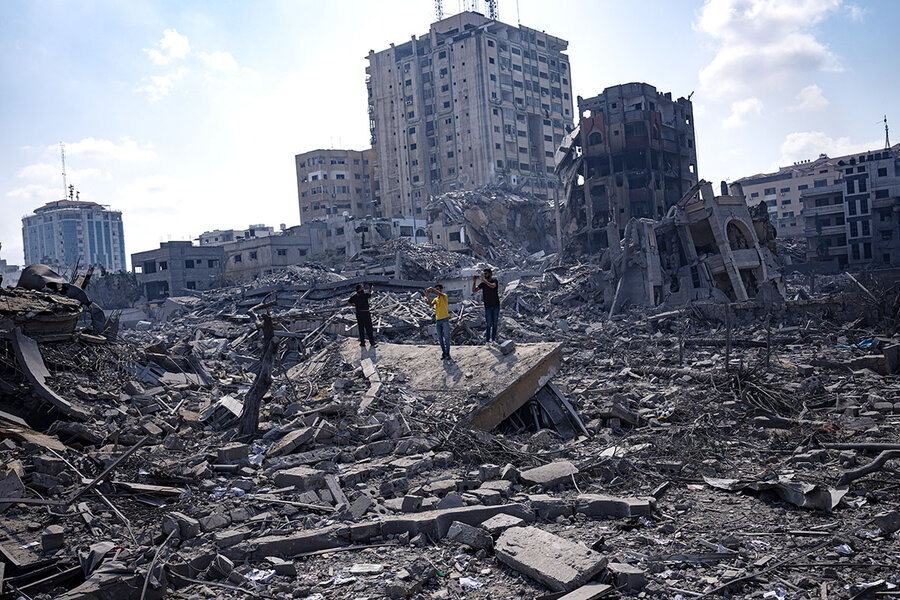The photograph depicts the aftermath of a severe disaster, possibly a bombing, as suggested by the extensive destruction in a cityscape. The area is thoroughly ravaged, with decimated buildings, vast piles of rubble, and a general sense of chaos and devastation. The city skyline is faintly visible in the background, though it offers little clarity on the precise location. Central to the image are three men, positioned atop what remains of a collapsed structure. Despite being small figures within the broader context of the scene, they draw attention as they appear to be documenting the destruction—likely by taking photos or recording video. Surrounding them are concrete chunks, blown-out windows, scorched shrubs, and a leaning concrete structure in the foreground. The entire scene is enveloped in a gray, bleak atmosphere, emphasizing the severity of the event that transpired.